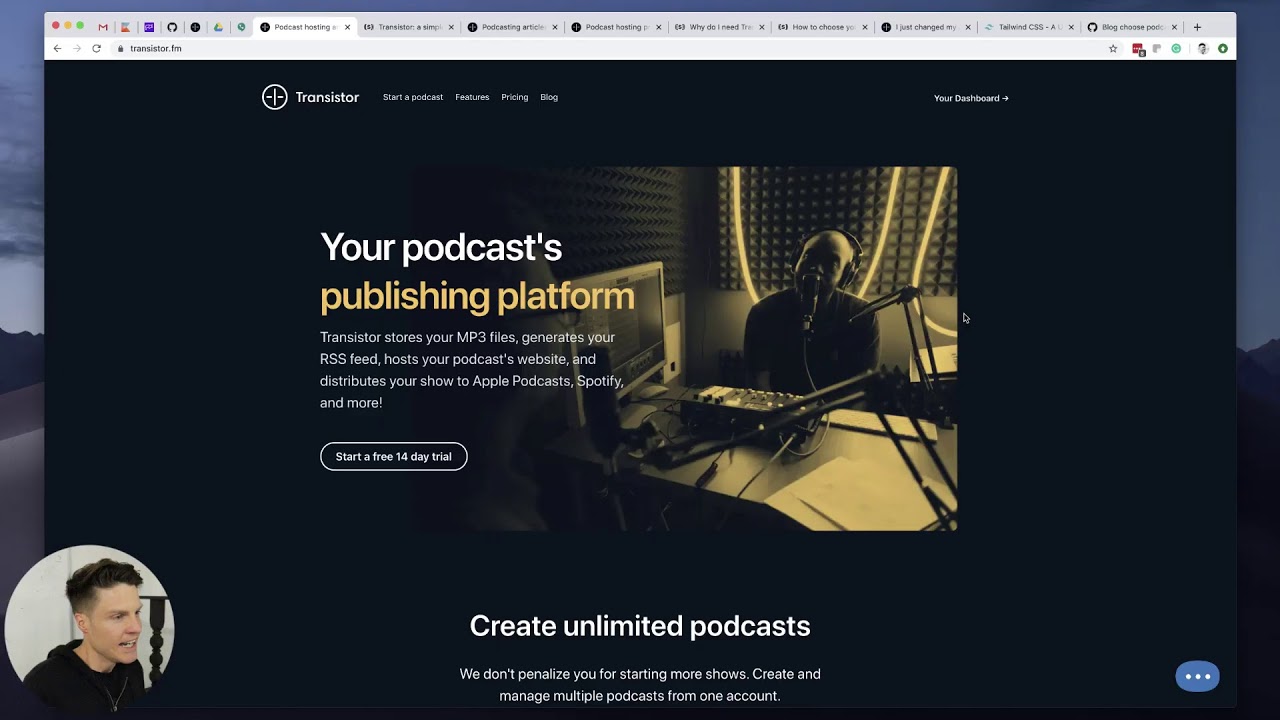The image is a screenshot taken from someone's computer, showcasing their desktop home screen with a spacious layout. The background features a serene sky at the top, transitioning to vibrant trees and lush grass at the bottom. 

Dominating the screen is a web browser window with multiple open tabs, distinguished by a gray border at the top and a black background beneath it. The active tab displays a website for 'Transistor,' a podcast publishing platform. The site's logo, a white circle with a vertical line flanked by dashes, is prominently displayed. Below the logo, the navigation menu highlights sections such as "Start a Podcast," "Features," "Pricing," and "Blog."

The main content showcases an image of a man wearing headphones, speaking into a microphone with a computer in front of him. To the left of this image, bold text reads "Your Podcast Publishing Platform." A call-to-action button inviting users to "Start a Free 14-Day Trial" is also visible.

In the bottom left corner of the screen, a small circular pop-up features a Caucasian male with short black hair, sporting a black hoodie. The message "Create Unlimited Podcasts" is centered at the bottom, while the bottom right corner features a blue oval shape with three white dots, indicating an interactive element or chat function.